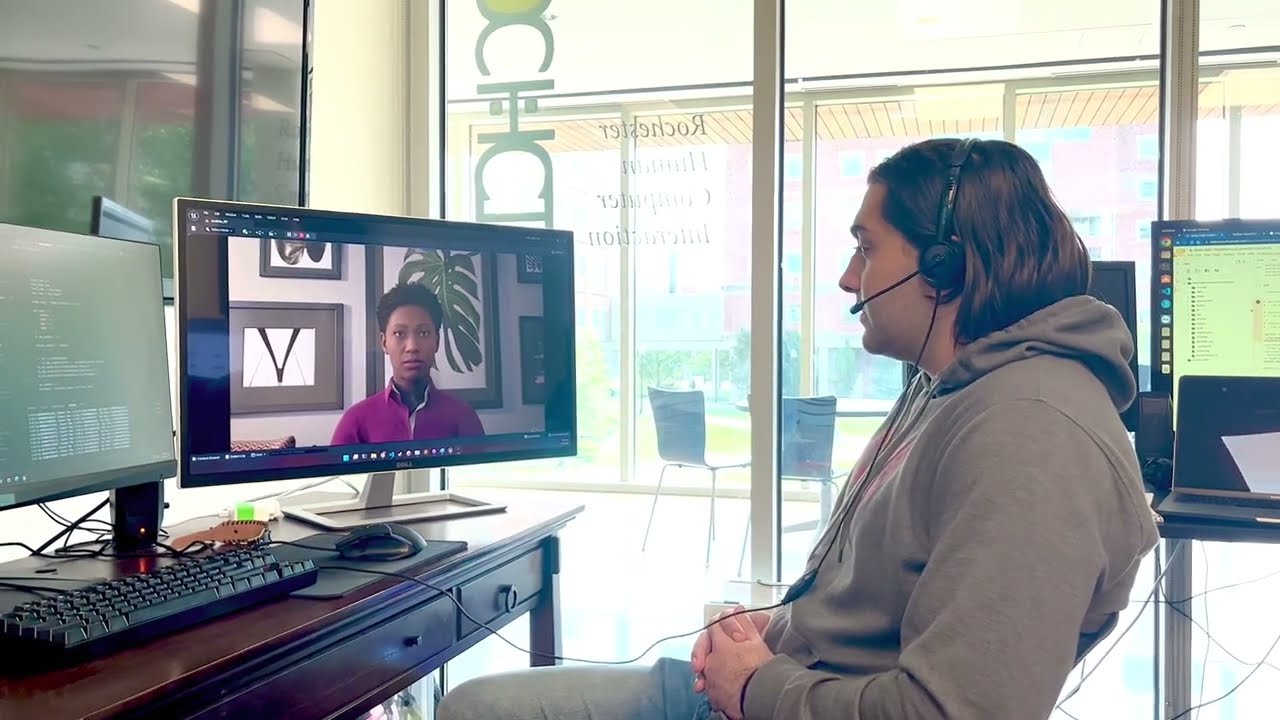In the image, a young man in his 20s with long brown hair is seated at a desk in an office setting. He wears a black headset and a brown or gray hoodie, and his gaze is directed towards two monitors on his left. One monitor displays a video call with an African-American woman in a magenta quarter-zip, seated in her office with green and black pictures behind her. The second monitor appears to show code or data. The desk holding the monitors is brown, and there is a black keyboard and mouse on it. To the right of the man are additional pieces of technology, including a laptop and another monitor. The background features large windows, allowing bright light to flood the space, and there are a few black chairs visible, suggesting an office or lobby environment. The scene conveys a typical workday involving remote communication and interaction with technology, possibly for a project involving artificial intelligence.